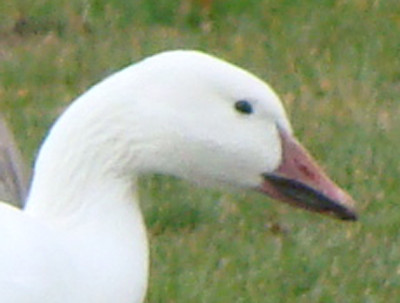This is a close-up photograph of a white goose in a green grassy field. The goose's head and part of its long, slightly curved neck occupy the center of the image, with its head positioned in a side profile. The goose has a small, beady black eye and a reddish-orange beak with a darker, almost black area around the mouth. The overall image quality is low resolution, making the background a blur of grass with some occasional brown patches, suggesting areas of dried or dead grass. Despite the blurriness, the goose appears alert and is clearly visible, staring intently towards the right side of the frame. The photo feels somewhat compact, emphasizing the goose's head and minimal surrounding details.